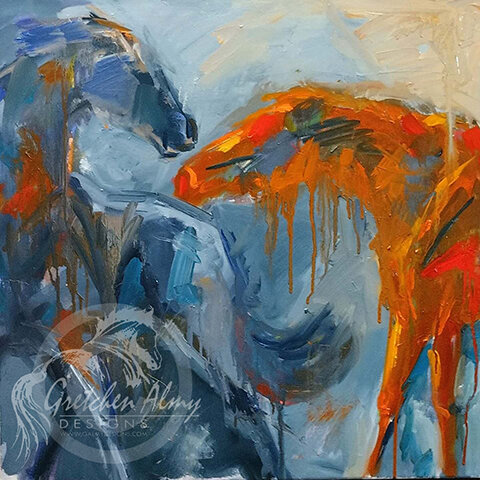This captivating impressionistic painting, attributed to Gretchen Alme Designs, vividly portrays two horses amidst a dynamic swirl of colors. Dominating the composition are an orange horse and a blue horse, their forms swathed in hues of orange, brown, red, light and dark blue, white, and gray. The horses are painted with fluid, dripping strokes that give the artwork a sense of movement and abstract beauty. The background is a blend of beige, bluish, light brown, and shadowy elements that add depth to the scene. In the bottom left corner, a cursive watermark reading "Gretchen Alme DESIGNS" in all caps forms a circular brand logo, subtly overlaying the art. The expertise and effort poured into this oil painting on canvas make it a mesmerizing piece to behold.